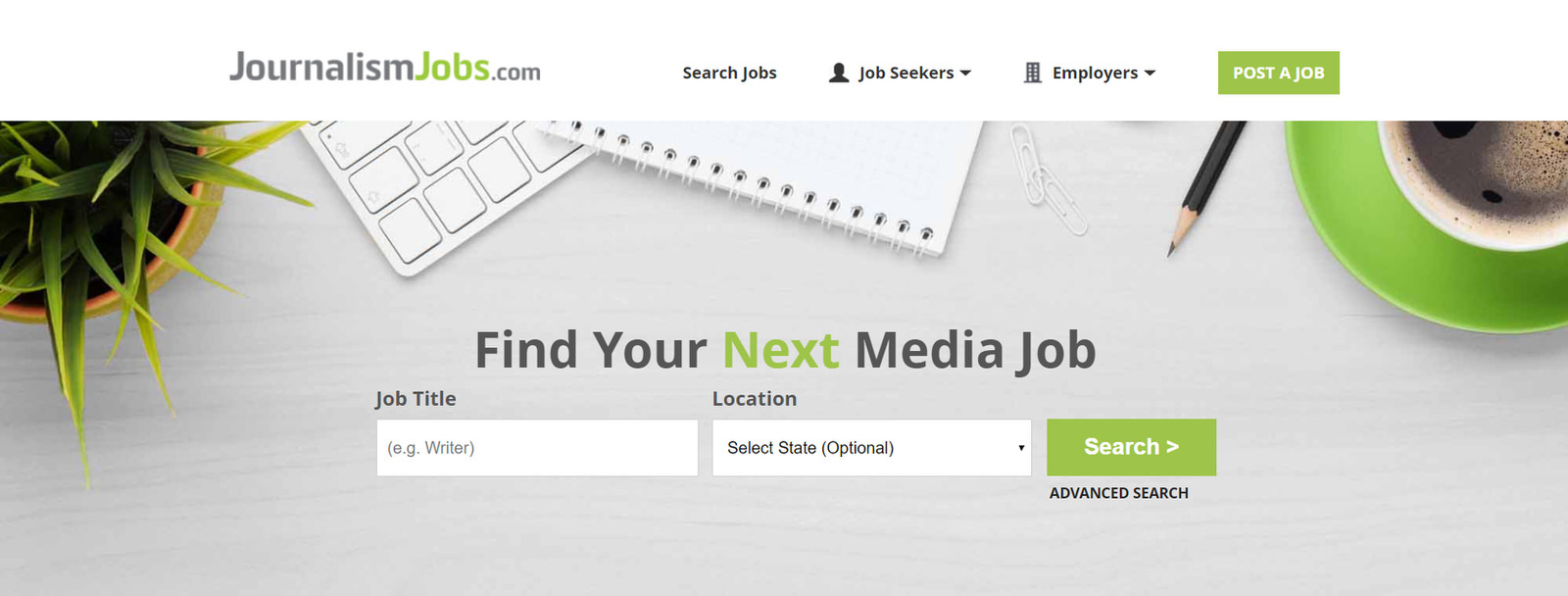This image is a screenshot of a webpage from JournalismJobs.com, featuring a sleek and professional layout. At the top, the page is predominantly white, showcasing the JournalismJobs.com logo. The word "journalism" appears in gray, "jobs" is highlighted in green, and ".com" matches the gray hue of "journalism." 

From left to right, the navigation bar includes options for "Search Jobs," "Job Seekers" (which has a drop-down menu), "Employers" (also with a drop-down menu), and on the far right, a prominent green button labeled "Post a Job."

Below this, there is an image depicting a tidy desktop setup. In the upper left corner of the image, there's a potted plant. Central to the arrangement is a keyboard and a notepad, with a pencil lying near them. There's also a coffee cup placed on a green coaster.

Centered on the page, a message in bold reads "Find your next media job," with the word "next" colored in the same green as the navigation button and the word "jobs" in the logo. Under this message are two white input fields: the first for entering a job title and the second, a dropdown for selecting a location by state, clearly marked as optional. Adjacent to these fields is a green "Search" button.

Towards the bottom of the display, there's an option for an "Advanced Search," offering more detailed search parameters.